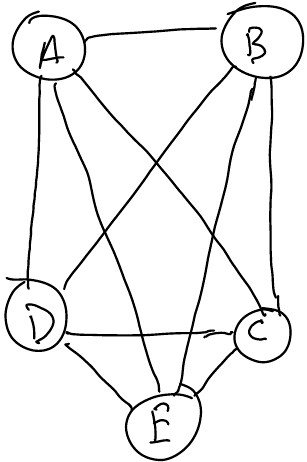This is a hand-drawn diagram illustrating the relationships between different components of a system. On the left side of the image, there's an incomplete circle labeled "A," from which four lines extend. The rightward line connects to another circle labeled "B," which slightly overlaps at its ends. Circle "B" also has four extending lines. One of these lines descends to the bottom of the image, connecting to circle "C," a fully drawn and complete circle. Circle "C" similarly has four lines emanating from it. One of these lines stretches diagonally downward to the bottom-right, meeting circle "E," a misshapen and incomplete circle with four lines of its own. Another line from circle "C" extends diagonally to the left, reaching circle "D." Circle "D" is mostly well-formed but has an errant line extending beyond its boundary. All five circles are interconnected, forming a complex network of lines which, at their convergence, create an upside-down five-pointed star.